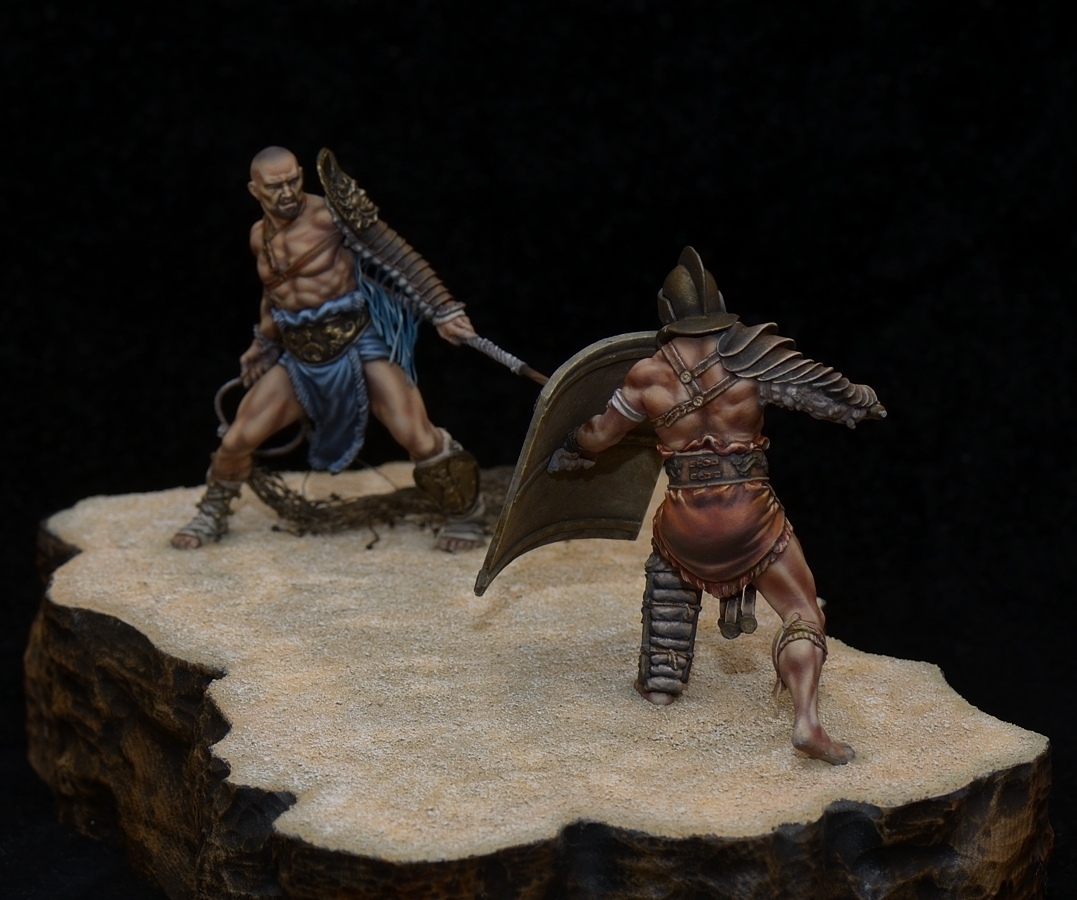The image is a detailed 3D illustration or potentially a hand-drawn art piece portraying two muscular male gladiators engaged in combat. Set against a stark black or void-like background, the fighters are depicted on a rocky, sandy terrain, evoking the feel of a small diorama. Both warriors wear tunics and heavily armored arm guards, extending up to their shoulders. 

The gladiator clad in blue sports an arm armor and wields a unique slashing rope weapon alongside a sword. In contrast, the other gladiator wears a brown material tunic and is equipped with a traditional Roman shield, a helmet, and both leg and arm protectors. Positioned in combat stances, they evoke the essence of ancient Roman gladiators, emphasizing their readiness and the intense atmosphere of their duel.